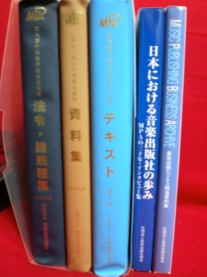In this photograph, we see five books standing upright against a vivid red background, arranged from left to right. Each book spine displays text primarily in Japanese, except for the far-right book which has English text reading "Music Publishing Business Archive." The leftmost book has a blue binding with "MR" at the top and is thin, wrapped in some kind of plastic. The second book features a yellow binding also reading "MR," and is slightly thicker with white Chinese characters. The third book has a light blue binding, "MR" at the top, and is the tallest and heaviest with gold print on the side. The fourth book is a darker blue with white Japanese symbols. The fifth book is greyish-blue, possibly wrapped in plastic, and is slightly pinched at the bottom as if melted slightly. All the books appear to be well-arranged and similarly sized, standing upright on their edges with spines facing the observer.